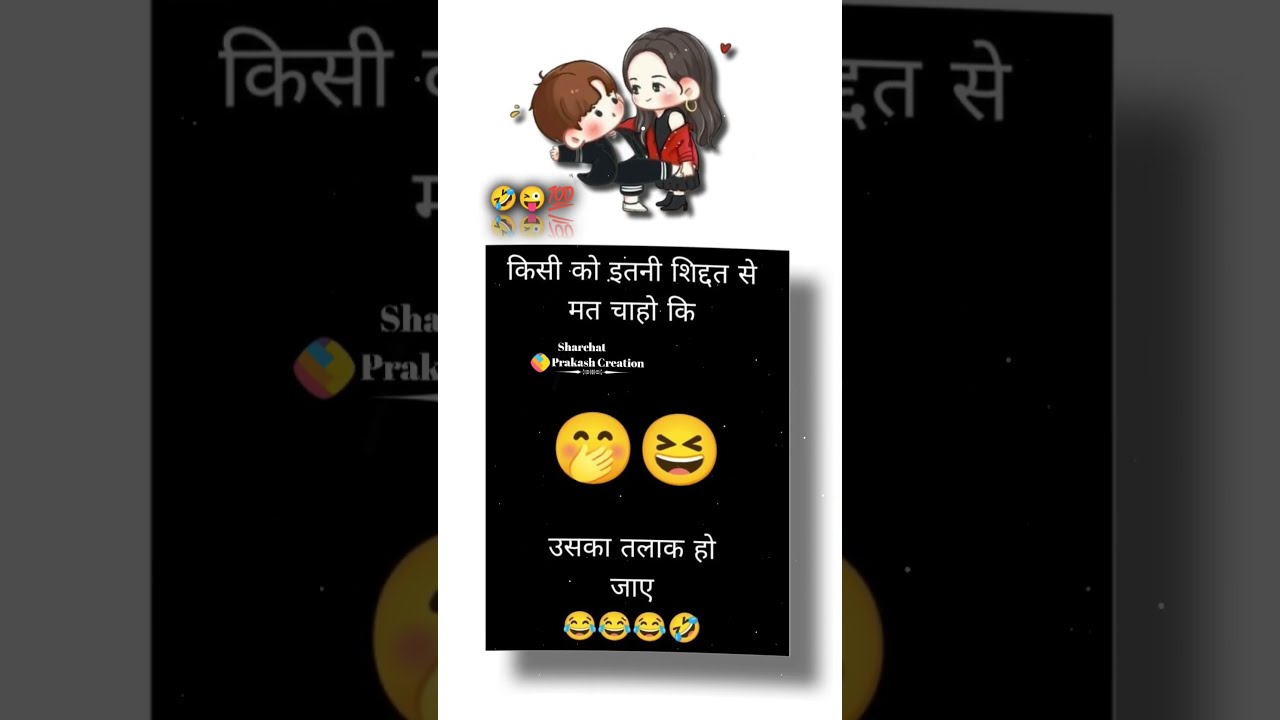The image depicts a screenshot that resembles a social media video post on a vertical phone screen, featuring an animated scene at the top. The upper portion showcases two anime-style characters—a boy and a girl—who appear to be dancing or in an embrace. The boy, with short brown hair, is dressed in a black outfit with a white t-shirt and shoes, and he has a light brown butterfly next to his head. The girl has dark brown hair, is wearing a black dress with a red sweater falling off her shoulders, black shoes, gold hoop earrings, and has a floating heart beside her head.

Above the characters, there are two yellow emojis on a white background: a laughing emoji with tears and a smiling emoji with its tongue sticking out. To the right, there's a "100%" emoji. Below the characters, written in white text, is "Prakash Creation," set against a black card-like background. The card also features some text in Hindi across the top. Below this, there are two emojis—a smiling face covered by a hand and a laughing face with tears. The bottom section of the image, possibly showing another post within the screen, contains more Hindi text and several laughing emojis with tears, including one at an angle. The predominant colors in the image include black, white, red, brown, yellow, gold, blue, pink, and orange, creating a vibrant, Instagram-style aesthetic.